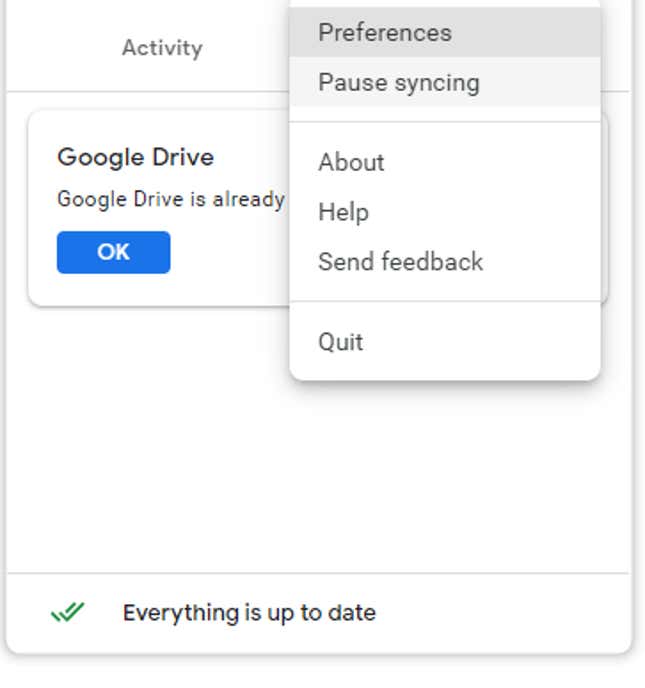A slightly blurry screenshot captures a moment within the Google Drive interface on a user's screen. Central to the image is a dropdown menu highlighting the "Preferences" option in darker gray, suggesting the user is about to select it. Below "Preferences," the options "Pause Syncing," "About," "Help," "Send Feedback," and "Quit" are visible, each separated by fine gray lines.

In the background, partially obscured by this menu, another section of Google Drive is visible with the text "Google Drive" prominently displayed, though additional text is unreadable. A bright blue "OK" button stands out amid the interface.

At the bottom of the screen, a double green checkmark icon accompanies the reassuring message, "Everything is up to date." To the upper left, a menu labeled "Activity" can be seen, bordered by light gray lines that separate it from other interface elements. All menus and pop-up windows exhibit a design with rounded corners and a slight shadow, adding a touch of smoothness and modernity to the overall layout.